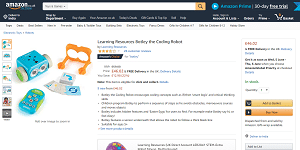This image is a small product listing on Amazon for a children's educational toy set. The set appears to be designed to encourage learning and imaginative play. It includes four distinct components: 
1. A small box on wheels adorned with googly eyes, giving it a playful, character-like appearance.
2. A deck of cards, likely used for educational purposes or games.
3. A remote control, possibly for interacting with one of the components.
4. A plasticky, orange headpiece resembling binoculars, which could be a learning tool or part of an interactive game.

The listing lacks clarity on the specific educational value or exact usage of the items. The price seems to be around $46. The interface shown is a typical Amazon product page, complete with "Add to Cart" and "Buy Now" buttons, additional images on the left, and an empty shopping cart indication on the top right.